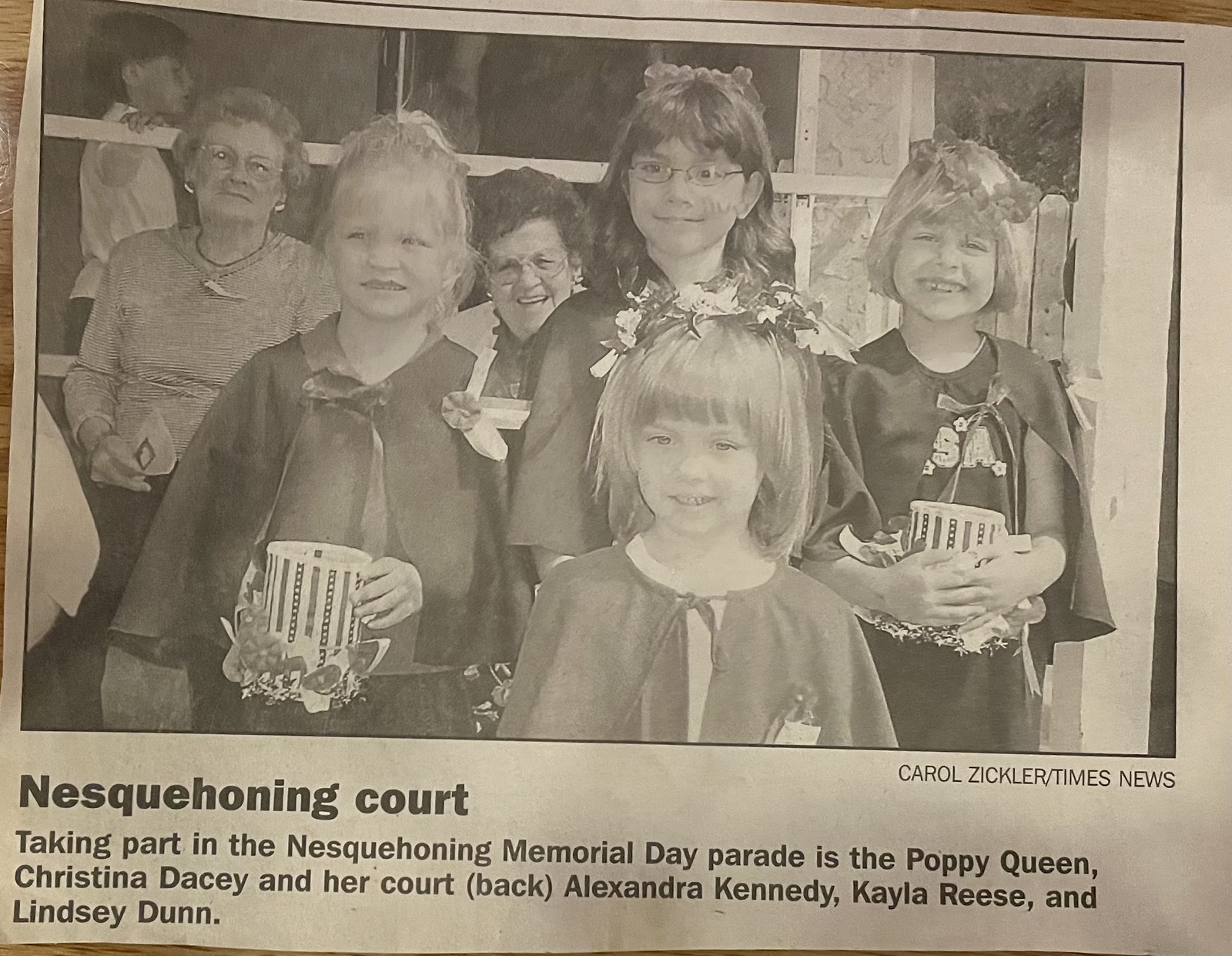This black and white newspaper clipping, now darkened with age, features a photograph capturing a nostalgic moment from the Nesquihoning Memorial Day Parade. At the forefront are four smiling young girls, each adorned with floral crowns and capes, holding what appears to be pots or large cups. Behind them stand two older women, also smiling, while further in the background, a small boy in a white button-up shirt leans against a rail, gazing at the scene. The topmost girl at the center, notably wears glasses. Below the image, the caption reads: "Nesquihoning Court, taking part in the Nesquihoning Memorial Day Parade, featuring the Poppy Queen, Christina Dacey, and her court: Beck, Alexandra Kennedy, Kayla Reese, and Lindsay Dunn." Additionally, it is credited to Carol Zickler, Times News.